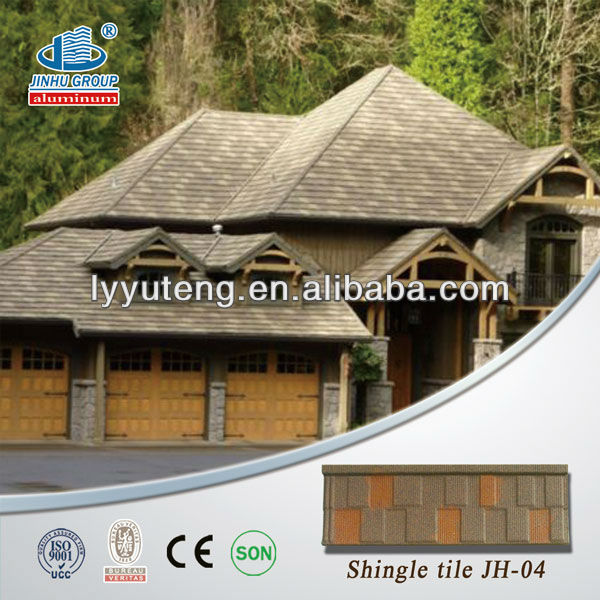The image showcases an elegant, expansive house likely used for a roofing advertisement. The house features a distinctive gray and white roof with multiple steep sections and numerous gables, highlighted by close-up details of the shingle tiles labeled "JH04" at the bottom right. The structure includes a three-car garage, a stately wooden front door under a small portico, and an upstairs balcony accented with wrought iron. Built predominantly from stone, with potential siding or wood sections, the house is set against a backdrop of lush green trees, suggesting a bucolic, forested location. In the top left corner, the name "Jinhoo Group" along with their registered trademark logo are prominently displayed in blue. Additionally, the middle of the screen features the web address "lyyuteng.en.alibaba.com," and several certification emblems, including ISO 900, Veritas, and others, are visible on the bottom left. The detailed and luxurious elements of the house, combined with the various logos and credentials, emphasize the quality and reliability of the advertised roofing materials.